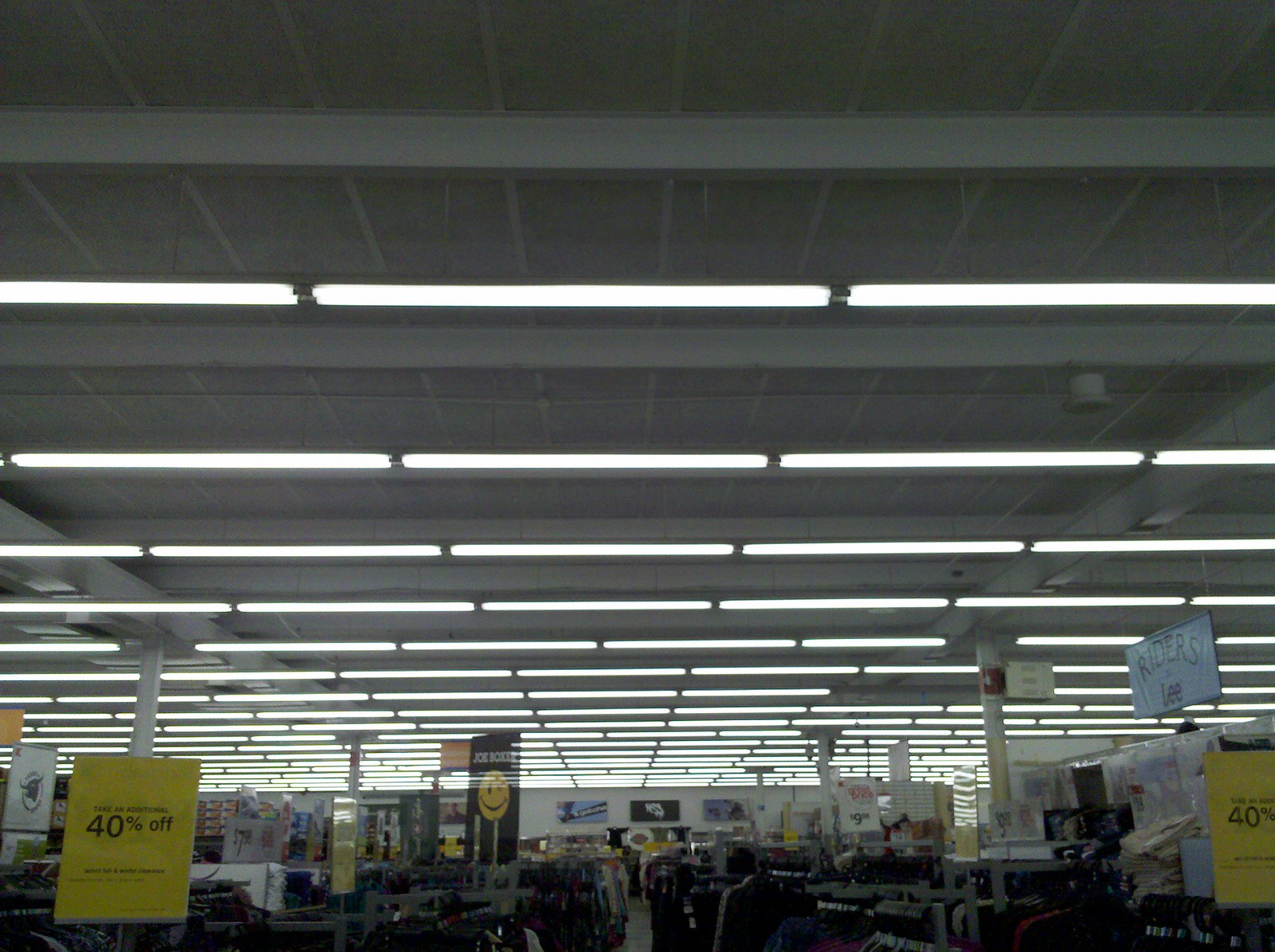This image captures the interior of a large retail store, possibly from 20 years ago, reminiscent of stores like Walmart. The focal point of the photo lies in the clothing department, dominated by racks upon racks of merchandise. Prominently displayed is a large banner featuring the Joe Boxer logo—a black background with "Joe Boxer" in white text and a large yellow smiley face. Additional signs indicate various brands, including one in the center that reads "Riders by Lee." Bright yellow sale signs adorn some of the racks, announcing 40% off discounts. The store's ceiling is lined with rows of fluorescent lights, casting a somewhat dim ambiance over the expansive space. Among the clothing, logos of sports teams like the Raiders can be discerned. In the far background, larger wall signs and a dressing room can be seen. Prices like $9.99 are visible on white signs, emphasizing the sale-driven atmosphere of this extensive retail environment.